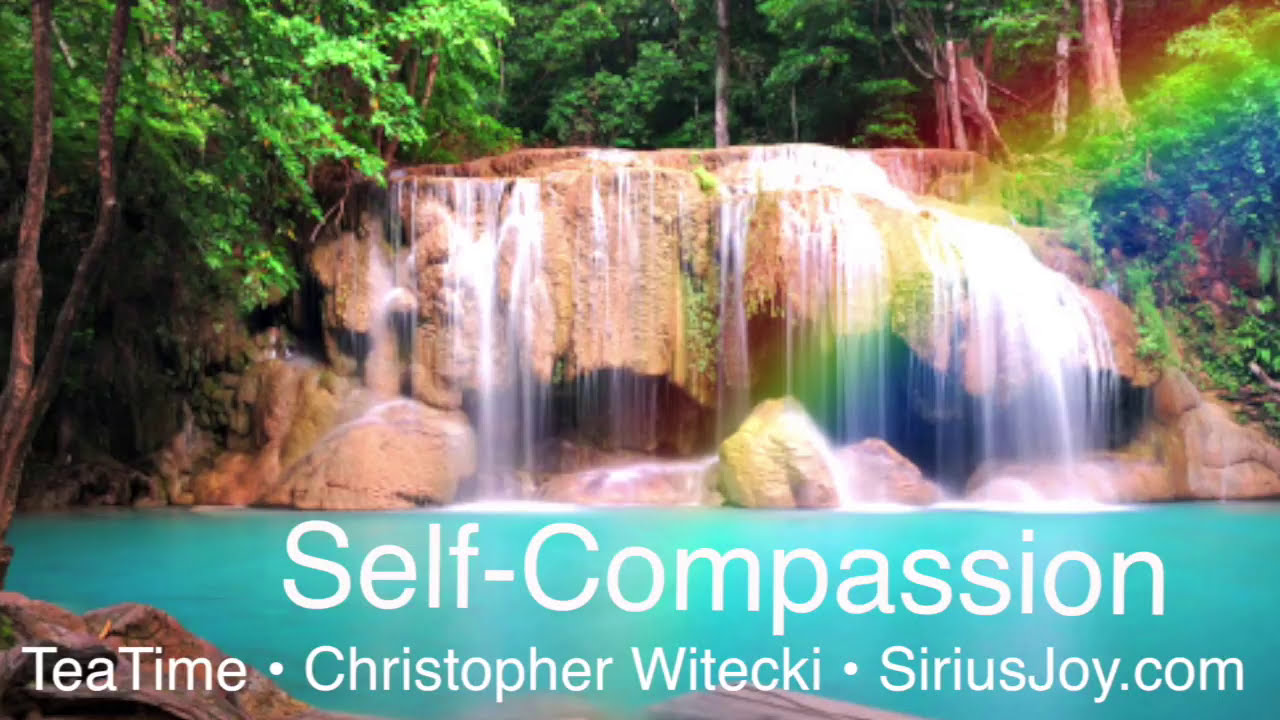The image captures a serene, natural setting featuring a modest waterfall approximately 10-15 feet high, located in a lush, densely forested area with rich green foliage and brown tree trunks framing the scene on the left, top, and right. Water cascades gently over light brown rocks into a bright blue pool below, creating a tranquil atmosphere. There is a subtle, possibly edited rainbow effect stretching from the upper right corner to the lower center, highlighting both the foliage and the flowing water. Adding to the imagery, a small cave is visible behind the waterfall, further enhancing the picturesque landscape. The bottom of the image displays text in white sans-serif font, which reads: "Self-Compassion." Below this, separated by dots, it continues with "Tea Time, Christopher Witecki, SiriusJoy.com," indicating that the image is likely a marketing asset for promoting an activity or service related to self-compassion, possibly counseling or an online community.